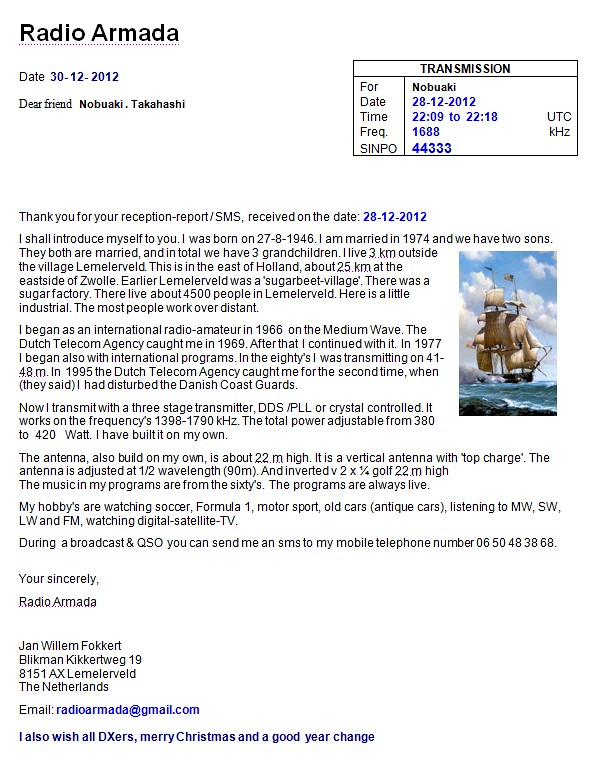The image displays a typed letter on a white background. At the top left, it reads "Radio Armada" with the date "30-12-2012." The letter is addressed to "Dear Friend, Nabuaki Takahashi." A rectangular box to the left details a transmission receipt for Nabuaki, dated "28-12-2012," with the time "2209-2218 UTC," frequency "1688 KHz," and SINPO "44333."

The letter begins by thanking Nabuaki for his reception report and SMS received on "28-12-2012." The writer, Jan Willem Folkert, introduces himself, mentioning his birth date "27-8-1946." He shares that he was married in 1974, has two sons who are both married, and collectively has three grandchildren. He lives three kilometers outside the village of Lemmerveld, which is in the east of Holland.

On the right side of the letter, there is an image of an old ship set against a blue sky with white clouds. The letter goes on for several paragraphs before concluding with "Sincerely, Jan Willem Folkert." Below this, contact information is provided: Jan Willem Folkert, Bilkman, Kickertweg 19, 8151AX, Lemmerveld, The Netherlands, and the email address RadioArmada@gmail.com.